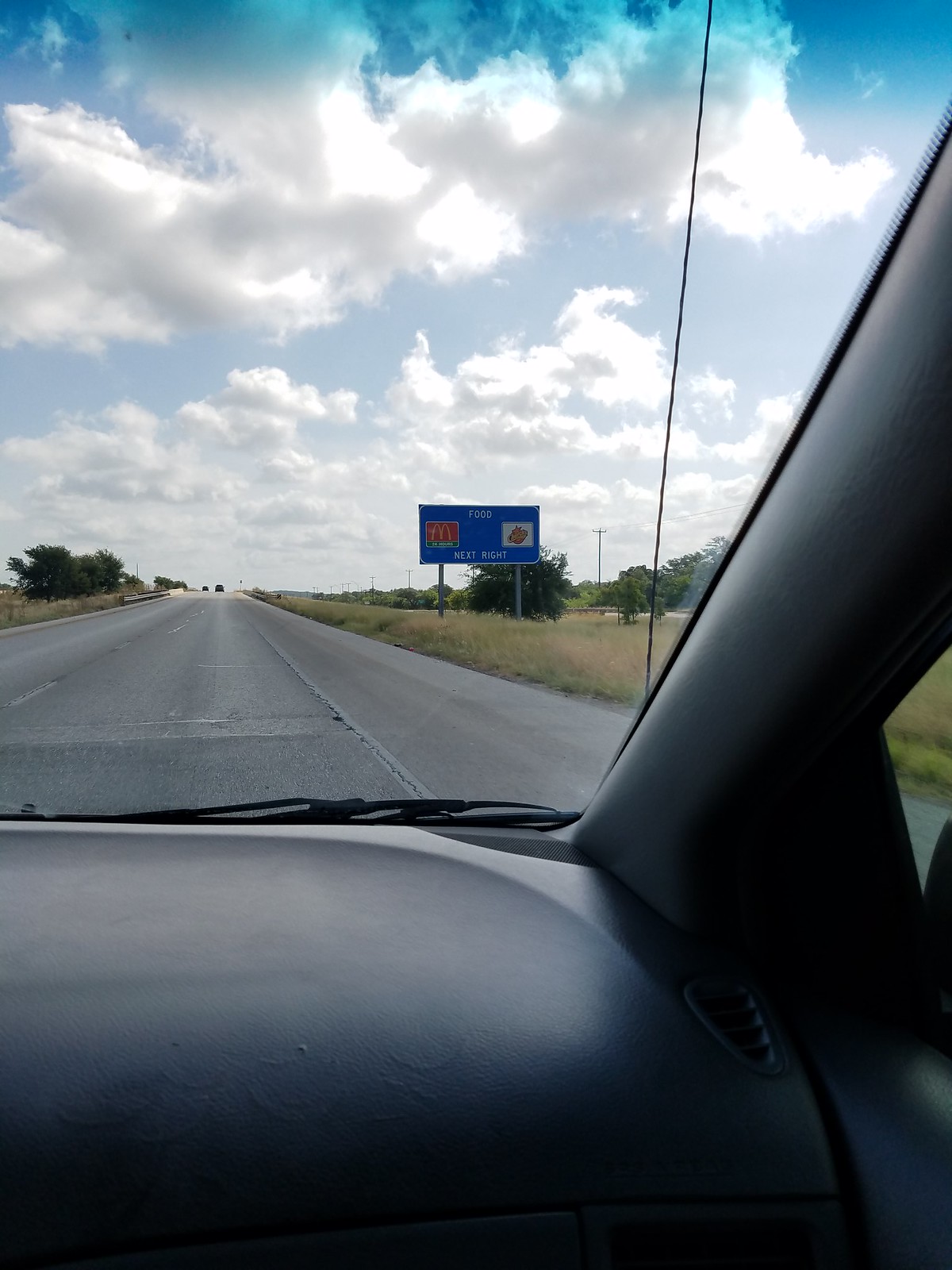A photograph taken from inside a car on a two-lane road, viewed from either the passenger or driver's seat. The car’s interior features a black vinyl dashboard and black plastic paneling around the windshield, with inactive black windshield wipers and an antenna extending vertically. The exterior scene reveals an overcast sky filled with well-lit cumulus clouds against a blue backdrop. The asphalt road, marked by a white dashed line in the middle and a solid white line on the right, gently rises into the distance, with a couple of trucks visible near the horizon.

On either side of the road are grassy areas, mostly yellow with some dry brushes and patches of green trees further away. To the right, there is a divider with tall, green, and brown grass, and nearer the road, a blue informational highway sign indicating "Food Next Right" with a familiar red McDonald’s logo and another logo, presumably for Church’s Chicken, featuring a white background and partially obscured details. On the left side, more trees and open grassy fields extend outwards, completing the serene landscape.